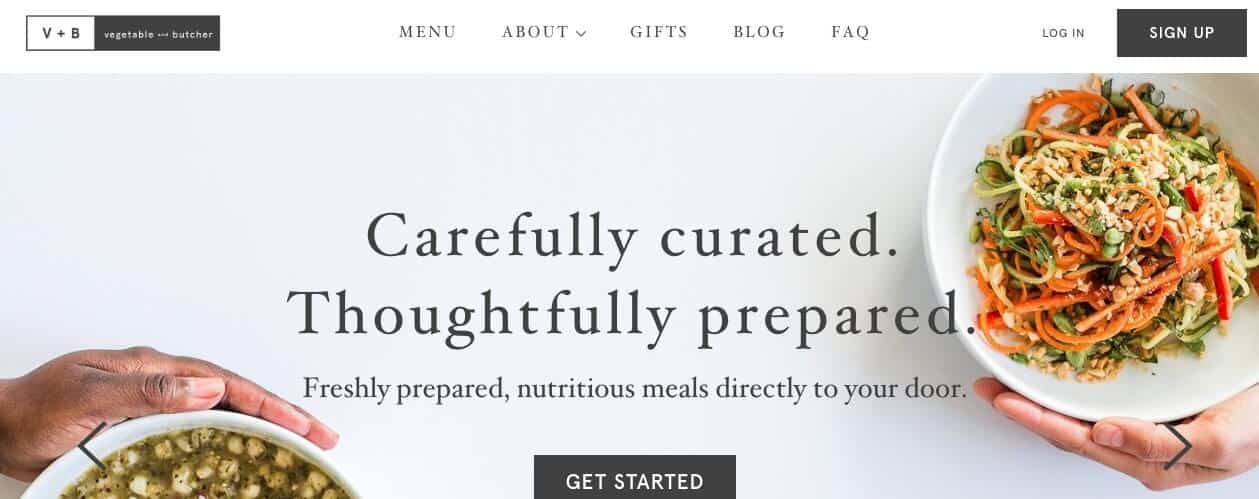The webpage's homepage is divided into two main sections. At the top is a sleek navigation bar, which includes a small box on the left: the left part of the box features a white background with black text reading "V + B," and the remaining two-thirds of the box has a black background with white text that reads "Vegetable and Butcher." Centered on the navigation bar are links directing to various sections of the website: "Menu," "About" (with a dropdown arrow), "Gifts," "Blog," and "FAQ." Towards the right side, you'll find black text that says "Login," next to a black square with white text that reads "Sign Up."

Below the navigation bar, the main splash screen features a visually appealing photograph. In the foreground, a white person’s hands are shown holding a colorful, green, orange, and white pasta dish. On the bottom left side of the image, a Black person's hand is holding a bowl of green pea soup with white balls in it.

Centrally aligned over the image is a series of compelling text phrases: "Carefully Curated," followed by "Thoughtfully Prepared," and in much smaller text below, it says "Freshly prepared, nutritious meals delivered directly to your door." At the very bottom of this section, there is a black box with white text that says "Get Started."